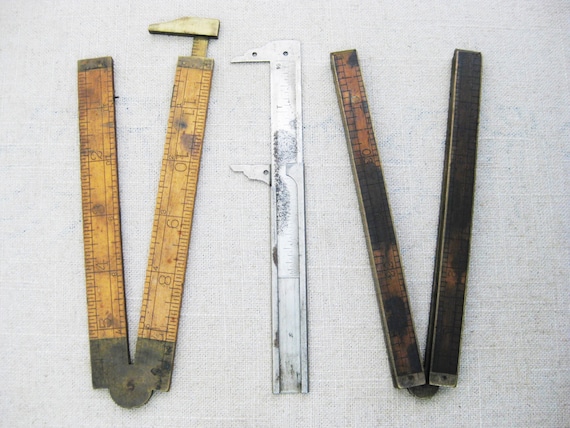This top-down color photograph showcases three distinct measuring tools arrayed horizontally on a light gray, canvas-like tabletop. On the left is a well-used, light brown folding wooden ruler with brass ends and a slider for measurements. It's folded into a V-shape and exhibits noticeable wear with black and gray smudges. The center features a slightly longer, stainless steel slide rule that appears metallic silver with some smudging, lying flat with its notches and indicators clearly visible. On the right, there is a darker brown wooden folding ruler, also in a V-shape, which is narrower than the left one and heavily covered in black smut. All tools have measurement notches and are approximately 12 to 16 inches in length when straightened. The overall composition on the neutral canvas backdrop highlights the functional and rugged nature of these architectural tools.